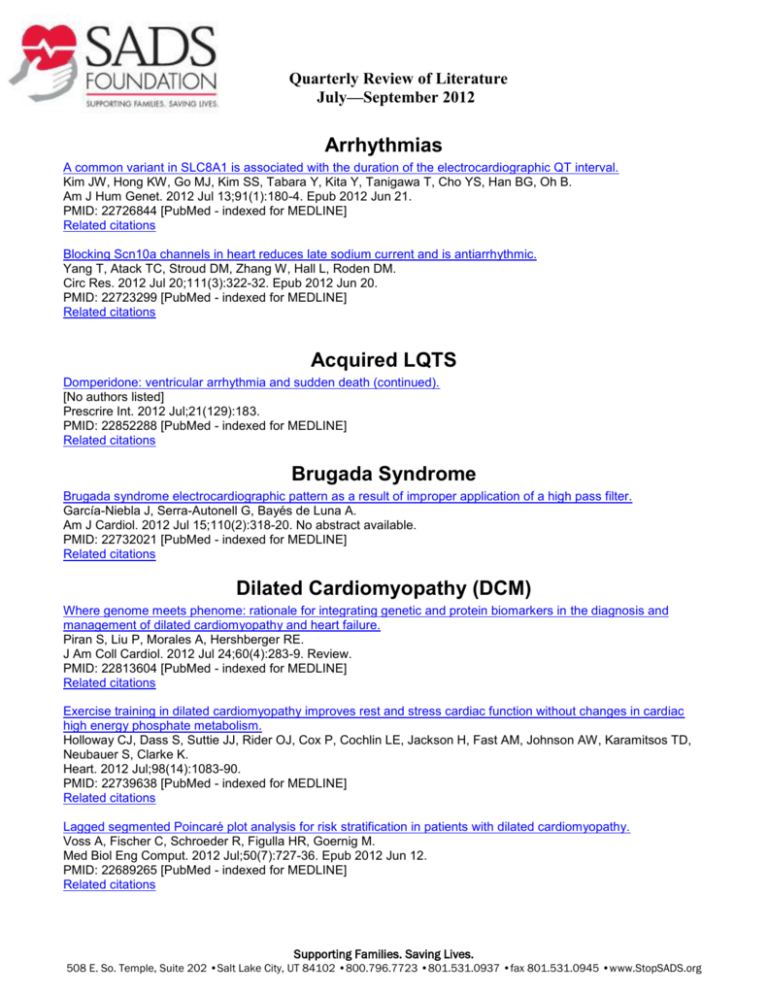This image is a document titled "Quarterly Review of Literature July to September 2012," featuring content extensively molded with blue hyperlinked text. In the upper left corner, there is a logo depicting a heart with a cardiogram line running through it, cradled by a right hand underneath. The logo represents the SADS Foundation, with the tagline "Supporting Families, Saving Lives."

The document is organized into several sections:

1. **Arrhythmias**:
   - "A common variant of SLC8A1 is associated with the duration of electrocardiographic QT interval."
   - Below this, numerous names, numbers, and dates offer attribution and specifics.
   - "Blocking SCN10A Channels in Heart Reduces Late Sodium Current and is Antiarrhythmic," followed by further details.

2. **Acquired LQTS**:
   - Describes information about ventricular arrhythmia and sudden death.

3. **Brugada Syndrome**:
   - Contains detailed descriptions and links to related citations.

4. **Dilated Cardiomyopathy (DCM)**:
   - Divided into three main subsections:
       - "Where the Genome Meets the Phenome: Rationale for Integrating Genetic and Protein Biomarkers in the Diagnosis and Management of Dilated Cardiomyopathy and Heart Failure."
       - Contains additional in-depth details and links.
       - "Exercise Training and Dilation: How It Improves Rest and Stress."
       - "Lag-Segmented Point Care Plot Analysis," with further elaborative information and associated citations.

Each section is supplemented with related citations hyperlinked at the bottom left.